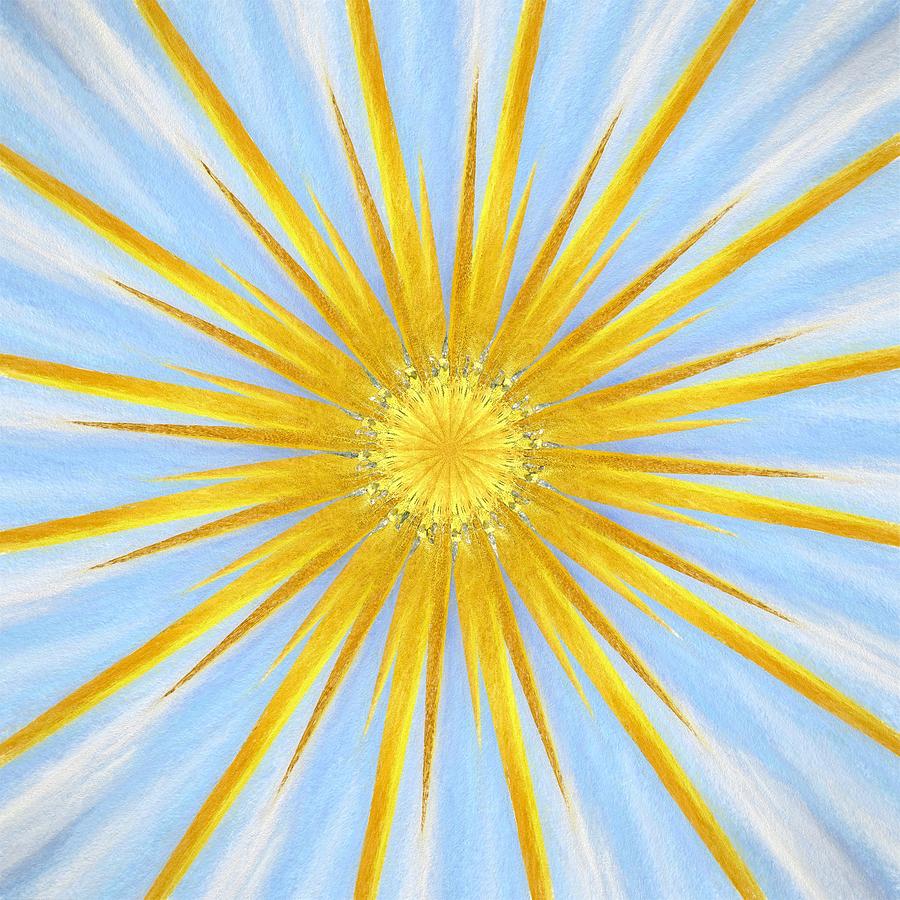This image features a highly detailed, close-up pastel drawing resembling a radiant sunburst or possibly the center of a flower. The background is a light blue with streaks of white extending vertically from top to bottom. At the very center lies a bright yellow circle, akin to the heart of a dandelion, featuring a subtle light brown interior. From this central point, variously hued rays emanate in all directions. The longer rays are predominantly a lighter, taxi-cab yellow with occasional shading, while the shorter rays take on a mustard-yellow tone. Some rays even extend further with shaded white light. The overall composition is two-dimensional, with a harmonious blend of blues, yellows, and whites, creating an image that simultaneously suggests the sun's vibrant energy and the delicate structure of a flower.